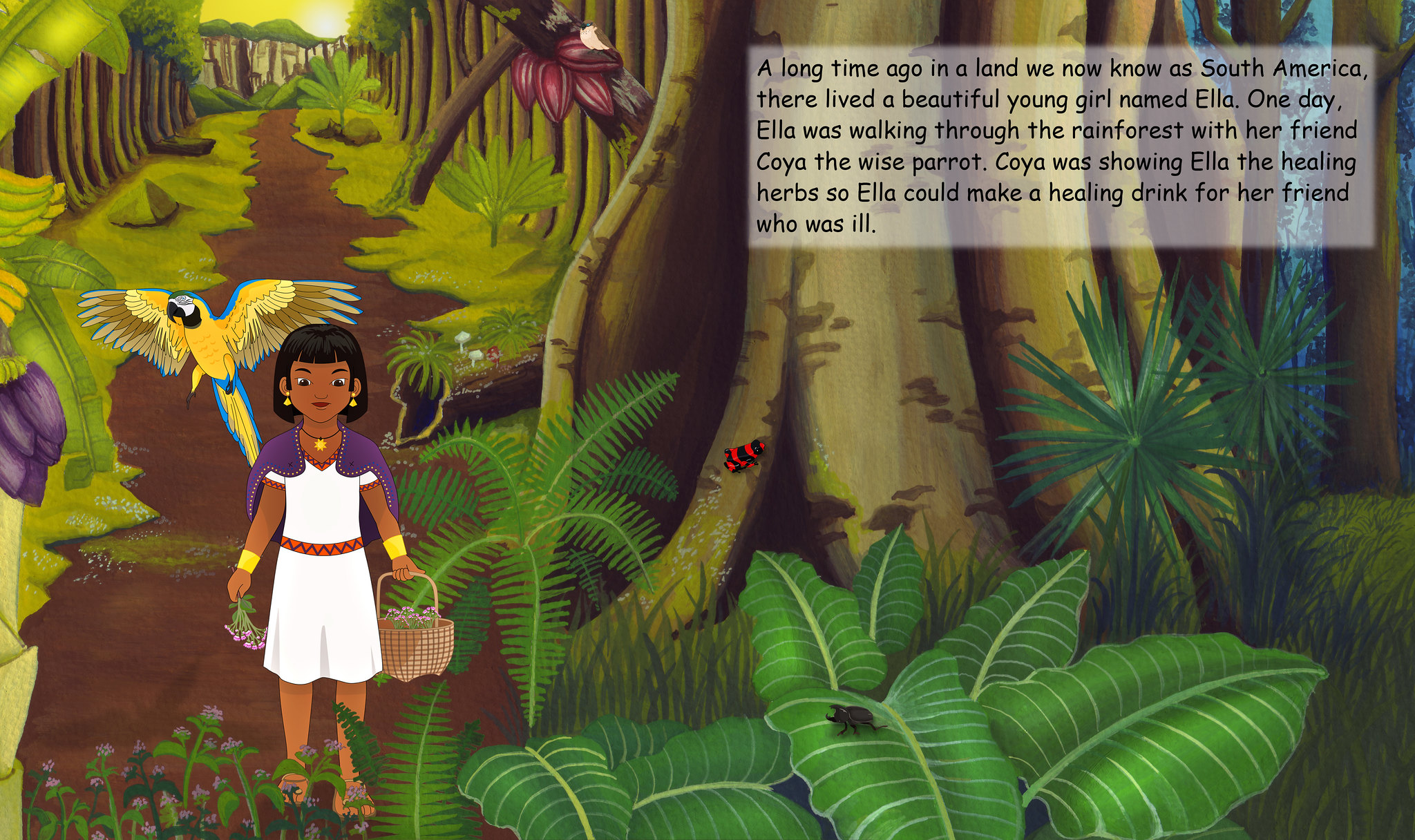The animated image depicts a vibrant rainforest scene from a long time ago in a land now known as South America. It features a beautiful young girl named Ella, who has darker skin and short dark hair with bangs, reminiscent of Dora the Explorer. Ella is wearing a white dress with a red belt and gold cuffs on her wrists as she walks along a path strewn with colorful flora. In her hands, she holds a small basket filled with flowers or herbs, while her wise parrot friend, Koya, a striking yellow and blue bird, flies just above her right shoulder. Together, they are gathering healing herbs to make a medicinal drink for an ill friend. The backdrop is lush with towering trees, ferns, and other vibrant plants, with the faintest glimpse of sky and sun in the background. The top right corner of the image bears the text: "A long time ago in a land we now know as South America, there lived a beautiful young girl named Ella. One day, Ella was walking through the rainforest with her friend Koya, the wise parrot. Koya was showing Ella the healing herbs so Ella could make a healing drink for her friend who was ill."